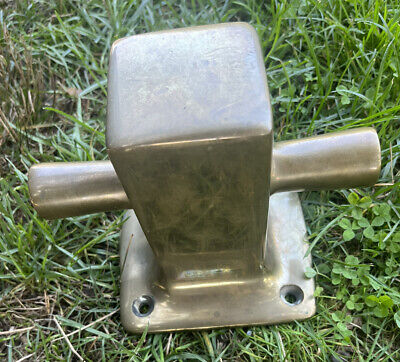This image, captured from above outdoors, depicts a vintage brass boat bollard post prominently situated in the middle of a verdant grassy area. The grass, characterized by its long, wispy blades and vibrant green hue, also includes a small patch of clover on the bottom right side. The bollard post, made of brass and primarily taking up the central portion of the image, features a substantial rectangular column at its core. Out from the left and right sides of this column extend two cylindrical, pole-like protrusions. The base of the bollard is a square, equipped with small holes at each of its front corners, presumably for screws. The overall composition highlights the striking juxtaposition of the antique metallic structure against the lush, green outdoor setting.